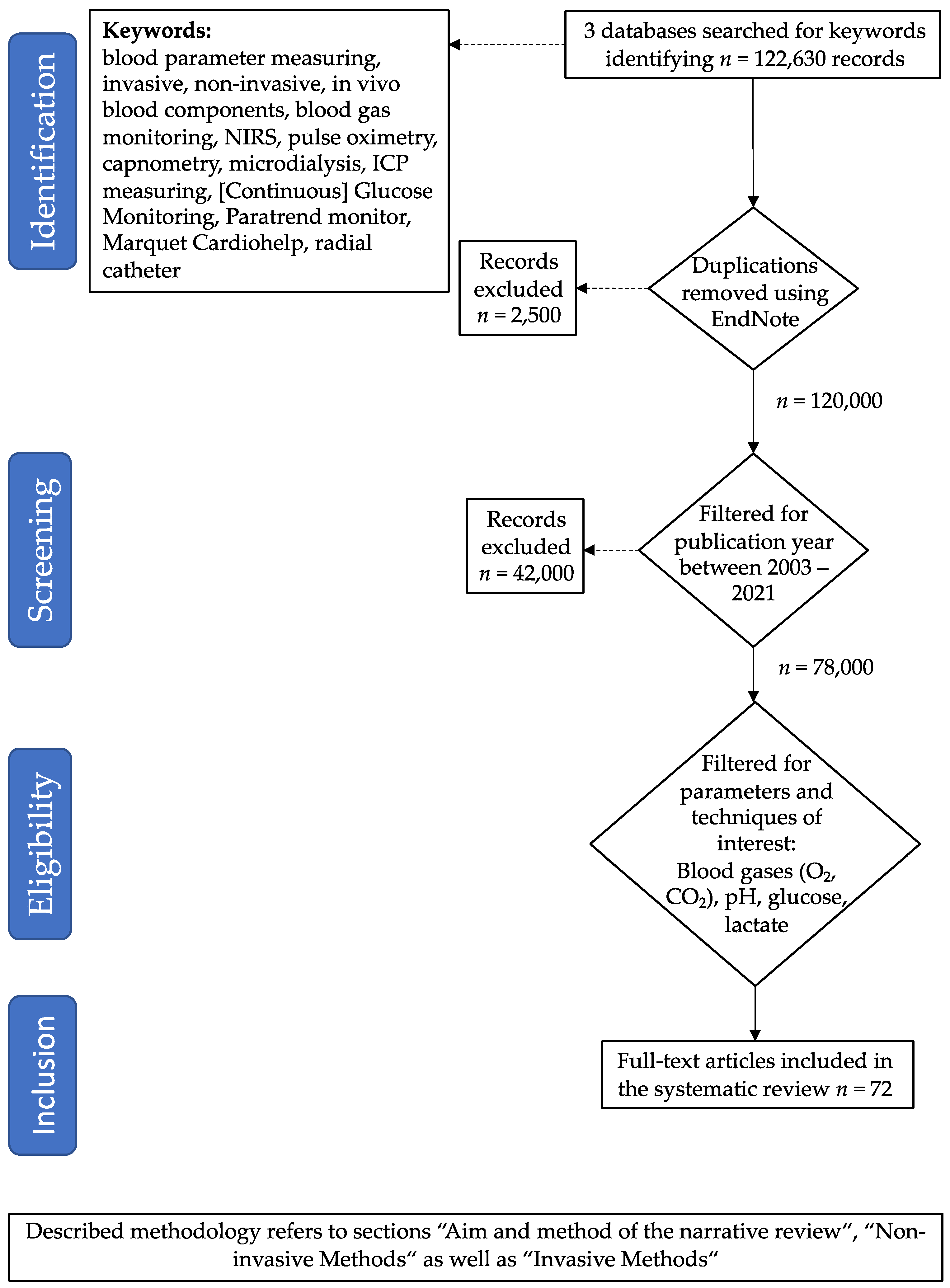The image is a detailed flowchart that outlines a systematic review process in a step-by-step manner. On the left side, from bottom to top, the flowchart includes the categories "Inclusion", "Eligibility", "Screening", and "Identification", each labeled in white font with a blue background. 

To the right of "Identification", the bolded term "Keywords" appears, followed by a list of related terms: blood parameter measuring, invasive, non-invasive, in vivo, blood components, blood gas monitoring, NIRS, pulse oximetry, capnometry, micro dialysis, ICP measuring, continuous glucose monitoring, paratransmonitor, Marquette, cardio help, and radial catheter. These keywords are enclosed in a black box.

Above the keyword box, a large rectangle states "three databases search for keywords identifying (N=122,630 records)," followed by a dotted arrow pointing towards the keywords box. Below this, a solid arrow leads down to a diamond labeled "dupications removed using EndNote," with a dotted line branching to a box labeled "records excluded (N=25,000)." Another arrow continues downward from "duplications removed," indicating "filtered for publication year 2003-2021" (N=120,000), branching off to another exclusion box (N=42,000).

The flowchart continues with a filtered step for parameters and techniques of interest, such as blood gases (O2, CO2, pH, glucose, lactic), leading to whole text articles included in the systematic review (N=72). Finally, at the bottom, a large rectangle states "describe methodologies refers to sections aim and method of the narrative review, non-invasive methods as well as invasive methods."

Overall, this flowchart visually maps out the screening process for a systematic review, from initial identification of keywords to the final inclusion of relevant full-text articles.